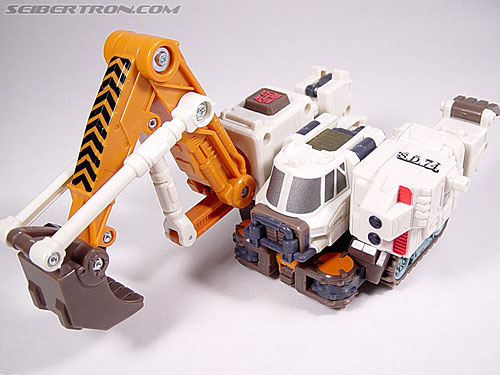In this detailed photograph, we see a toy excavator prominently displayed against a white or light gray background. The body of the excavator is primarily white with brown accents, particularly on the front. The machine is composed of three main sections: the engine, which is followed by the cab in the middle, featuring windows, and the crane extending from the right side of the cab. The crane's arm is orange and has two distinct joints, terminating in a brown scoop that matches the brown accents on the excavator's body. A notable feature on the crane is a brown button. The gray letters "Cybertron.com" are visible in the top left corner of the image, indicating the website where the toy can be purchased.